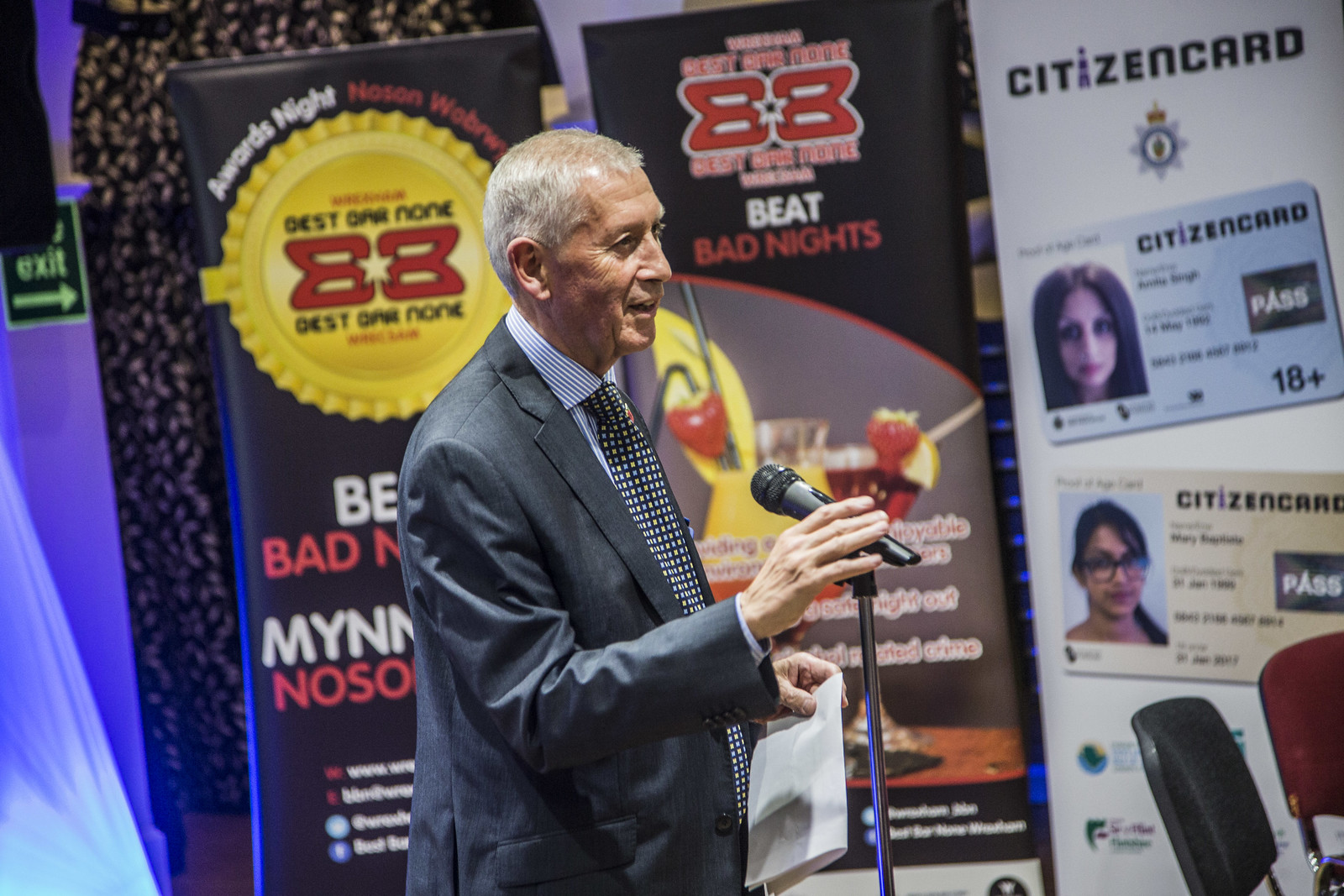The landscape-oriented color photograph captures an older man, identified as Erdogan Bilek, the president of Turkey, speaking into a standing microphone on stage at an expo or awards banquet. He has short, white hair and caramel-colored, slightly wrinkled skin. Bilek is dressed in a navy blue sports jacket paired with a light blue collared shirt and a black and white checkered tie. In his left hand, he holds a folded piece of paper. To his right, a white sign displays the words "Citizen Card" in black ink at the top, with several images of cards underneath, including a blue citizen card for an 18-plus girl with brown hair. The background features multiple tall banners, one of which has a large gold emblem with the words "Best Bar None 33." The scene includes chairs in front of him—a black one and a red one. The overall style of the image is photographic realism.